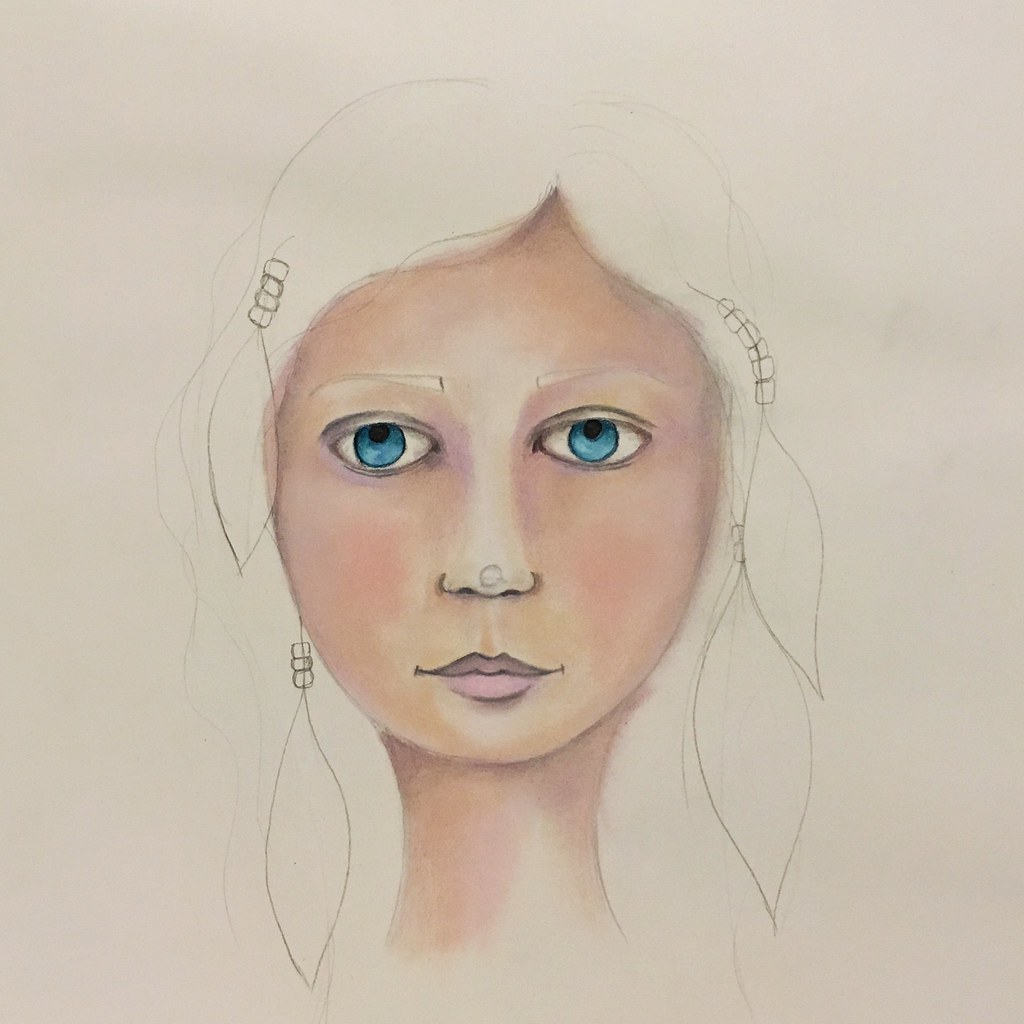This image showcases a work-in-progress drawing of a woman, primarily created with color pencils or possibly watercolor on off-white or light gray paper. The artwork is square-shaped with the woman's face centered on the sheet. The woman has striking blue eyes, pale skin with peach-tone shading, and pink lips accentuated with a stark lip liner. There is a notable circle on the tip of her thin nose, suggesting some form of jewelry. Her eyebrows remain penciled in but lack color. The hair, which is sketched and not yet painted, extends past her neck and includes feather-like shapes adorned with strings of beads above them. This part of the drawing is entirely in black and white. Shadows and slight accenting offer depth around her nose, lips, and eyes.